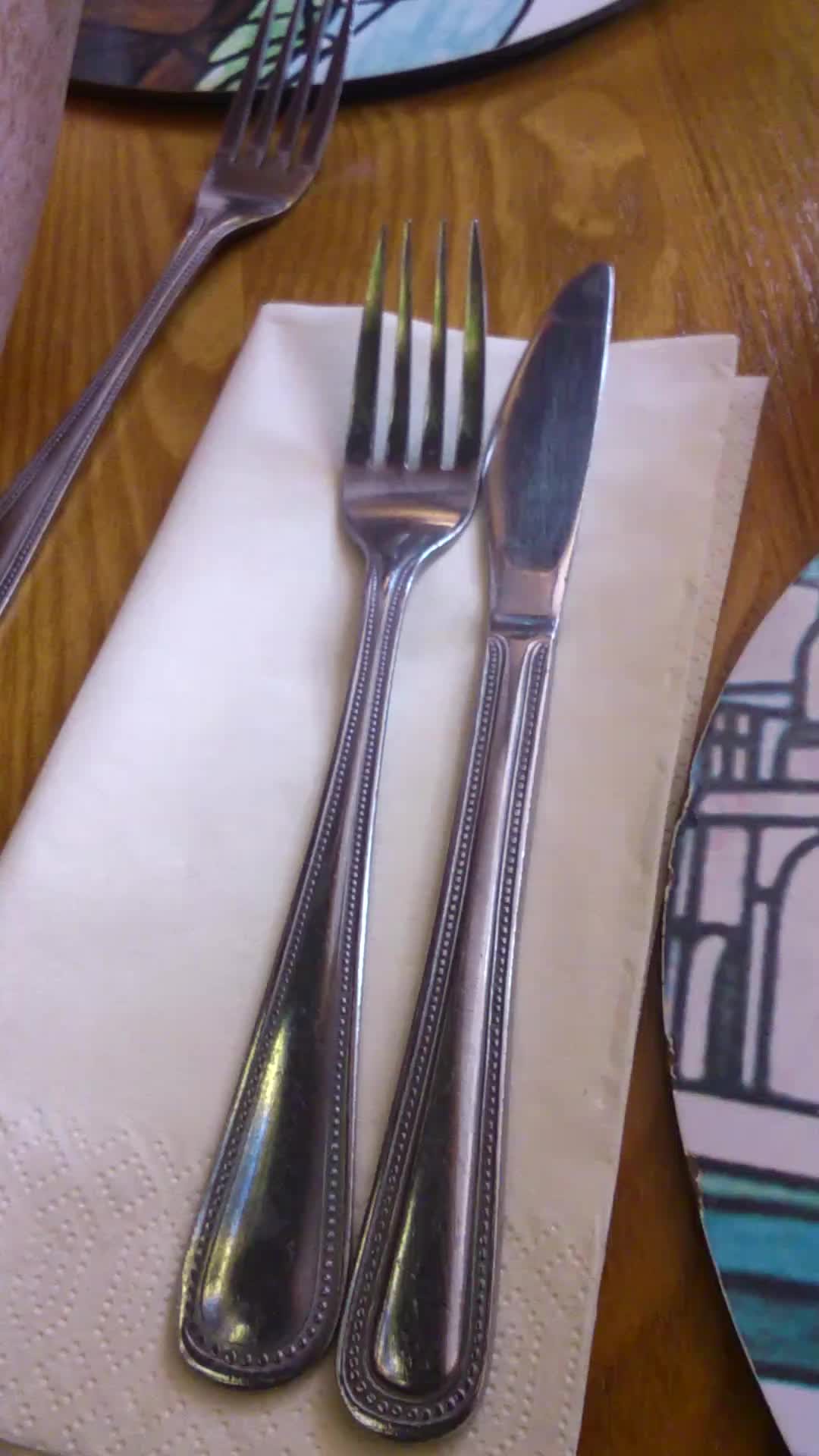This close-up photograph captures a carefully arranged place setting on a light brown wooden table. At the center is a folded white napkin positioned vertically, holding a reflective, light gray fork with four tines and a matching butter knife. Another fork, slightly larger, rests to the left of the napkin, partially touching the rim of a plate. The bottom right corner reveals the edge of another plate beside the napkin. Both plates feature intricate designs, including dark green, blue, black, and brown stripes and patterns, possibly depicting a cityscape or abstract shapes. The reflective silverware and detailed plate designs contrast beautifully with the natural wood grain of the table beneath.